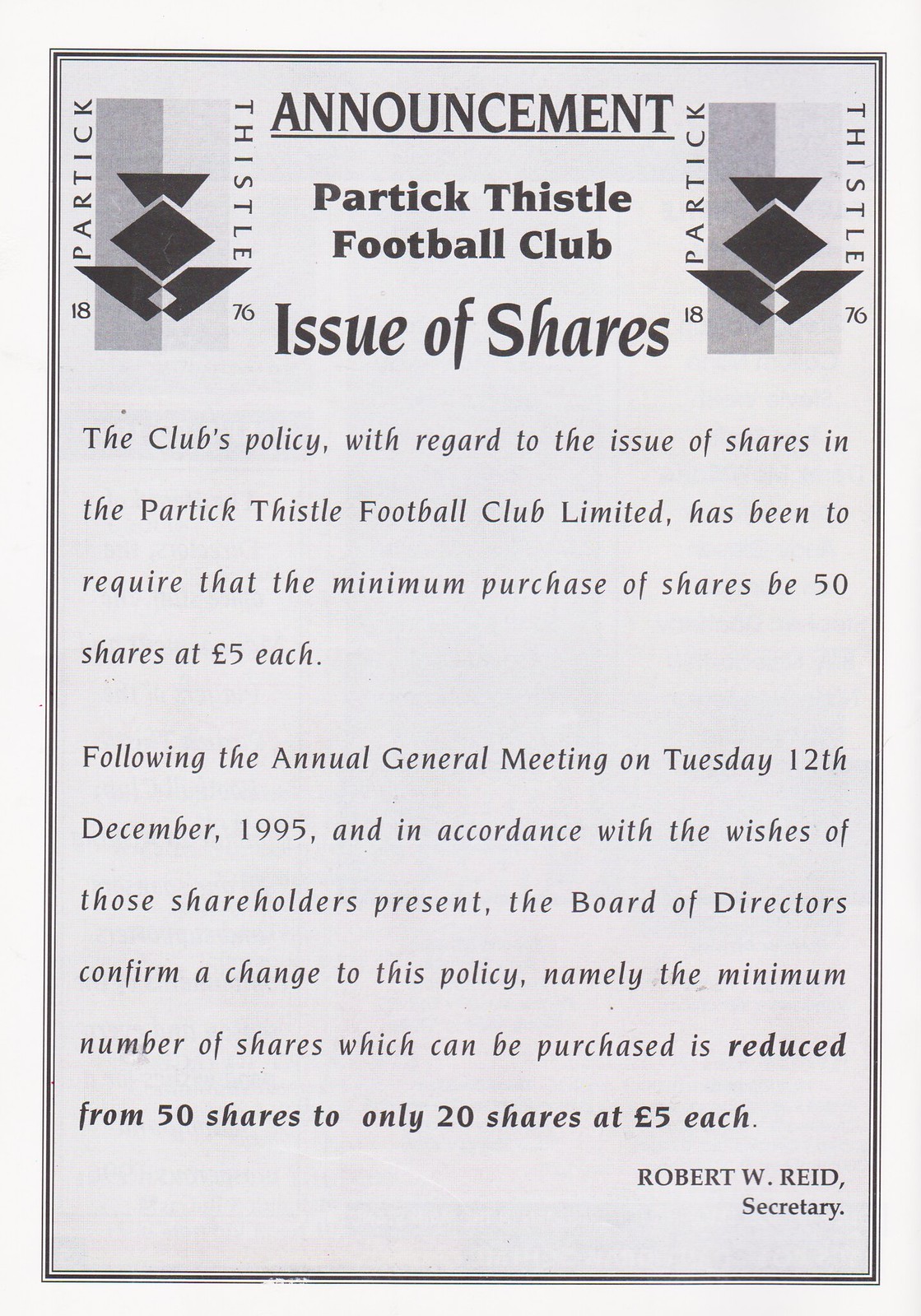This black and white scanned page, possibly from a football club program or flyer, features an announcement from Partick Thistle Football Club regarding a change in their share policy. The page has a decorative black border with the word "Announcement" at the top, flanked by Partick Thistle Football Club logos that include the year "1876" twice. The first paragraph states that the club's policy required a minimum purchase of 50 shares at £5 each. The second paragraph details a change following the annual general meeting held on Tuesday, December 12, 1995, where it was decided that the minimum share purchase would be reduced to 20 shares at £5 each, in line with stakeholders' wishes. The announcement is signed by Robert W. Reed, Secretary, in the bottom right corner.